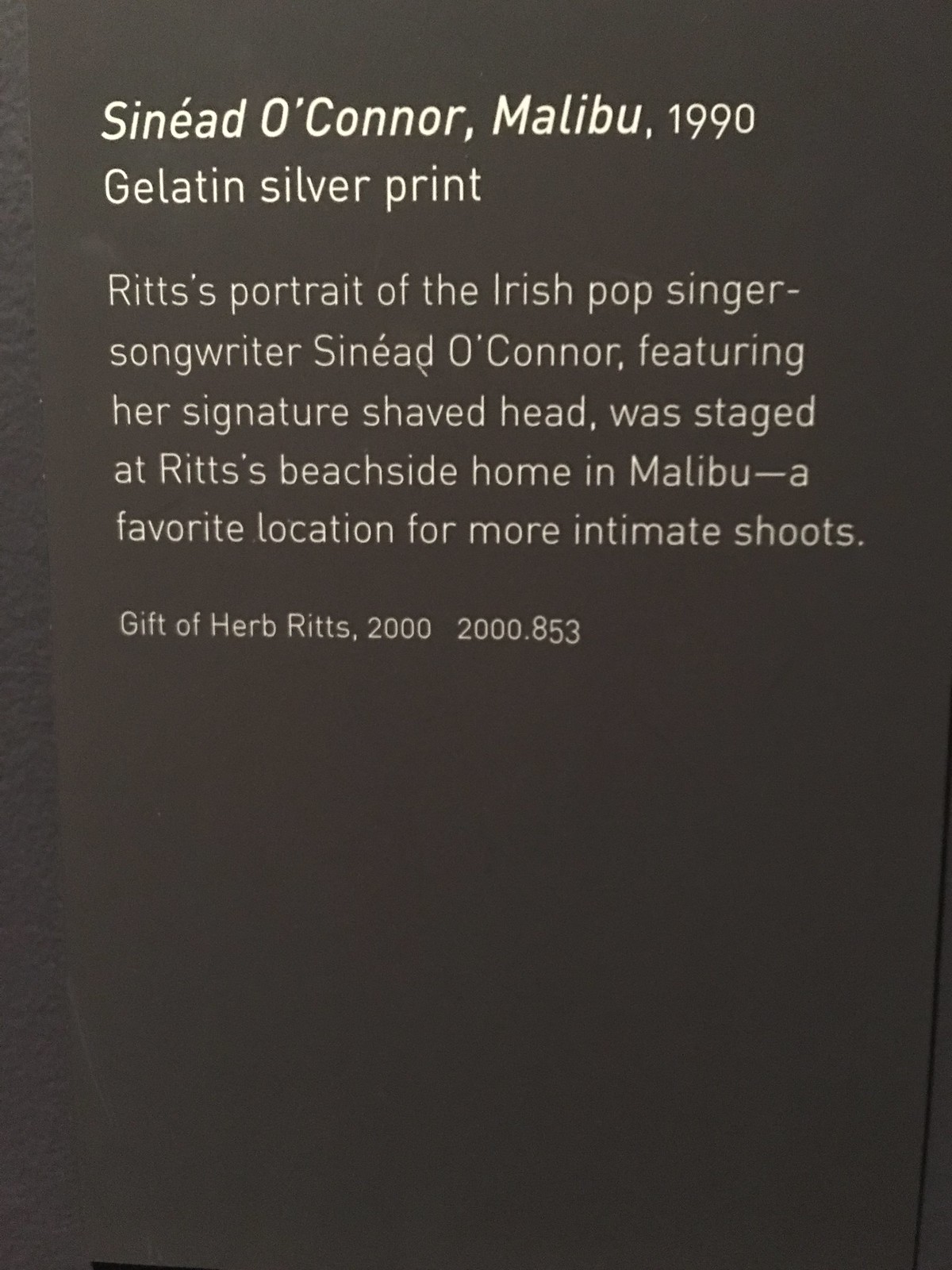The image features a placard with white text on a gray background. At the top, in bold and italicized white text, it reads "Sinead O'Connor, Malibu, 1990." Below that, in slightly larger non-italicized text, it states, "gelatin silver print." The main body of the text describes the piece: "Ritz's portrait of the Irish pop singer-songwriter Sinead O'Connor, featuring her signature shaved head, was staged at Ritz's beachside home in Malibu, a favorite location for more intimate shoots." The text concludes with, "Gift of Herb Ritz, 2000, 2000.853." The text's font size decreases progressively, with the final line being the smallest. This placard likely accompanies a photograph or artwork of Sinead O'Connor in a museum or private collection, providing context about the image and its origins.